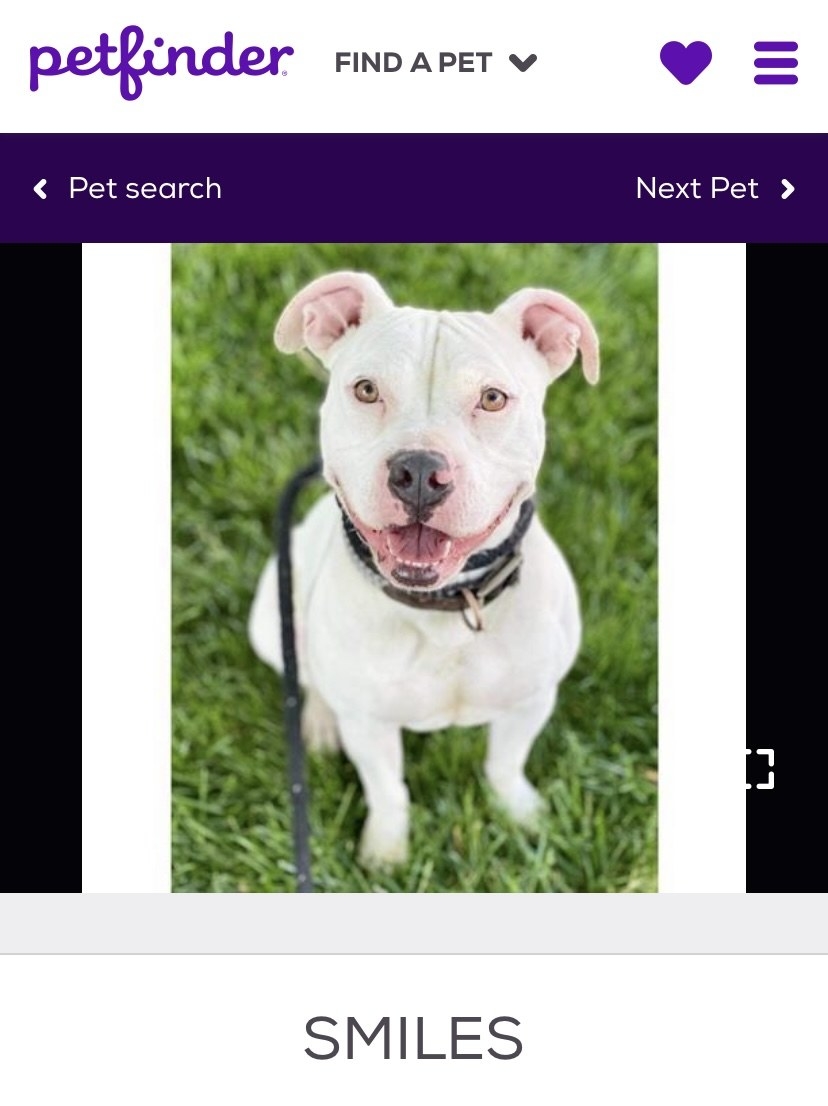This image appears to be a screenshot from a website, likely Petfinder. In the top left corner, "Petfinder" is written in elegant cursive lettering in a purple hue. Centrally located at the top of the image, there's a clickable button labeled "FIND A PET" in bold, uppercase black letters. To the right of this button, there is a clickable heart icon alongside three horizontal purple lines.

As you proceed downwards, a rectangular section in a dark purplish-black shade appears. At the top of this section, "PET SEARCH" is written, with a left-pointing arrow beside it. On the opposite side, there's a "NEXT PET" option with a right-pointing arrow.

Lower on the page, a photograph of a dog catches the eye. The dog is primarily white with small ears that curl down at the top. Its eyes are light-colored, and its mouth is open in what appears to be a smile, revealing a joyful expression. The dog is seated on a grassy area. Below this image, in large, bold, uppercase black letters, the word "SMILES" is prominently displayed.